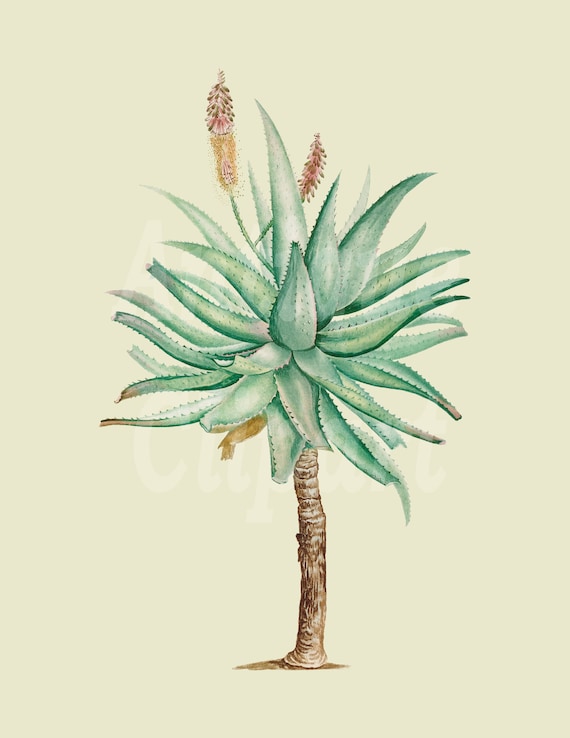The image is an intricate color illustration in portrait orientation that combines elements of both a succulent plant and a palm tree, presented as a botanical print. The centerpiece is a slender tree trunk with light brown bark, thin in stature yet prominently placed in the middle of the image. Its crown features an array of thick, jagged leaves that fan outwards, resembling the spiky, oval shapes typical of aloe vera leaves. Each leaf is rich green with white highlights that accentuate their teardrop-shaped pointed tips.

A distinctive aspect of the illustration is the presence of two red-flowered spikes emerging from the top. These are elongated, wheat-like flower structures with elliptical shapes, one leaning to the top right and the other more centrally positioned. They add vibrant detail to the plant's appearance. The background is a solid cream color, which provides a neutral backdrop and enhances the botanical focus of the artwork. Additionally, a barely legible white watermark runs across the center, subtly marking the illustration. The overall scene captures the essence of botanical art, blending naturalistic detail with creative interpretation.